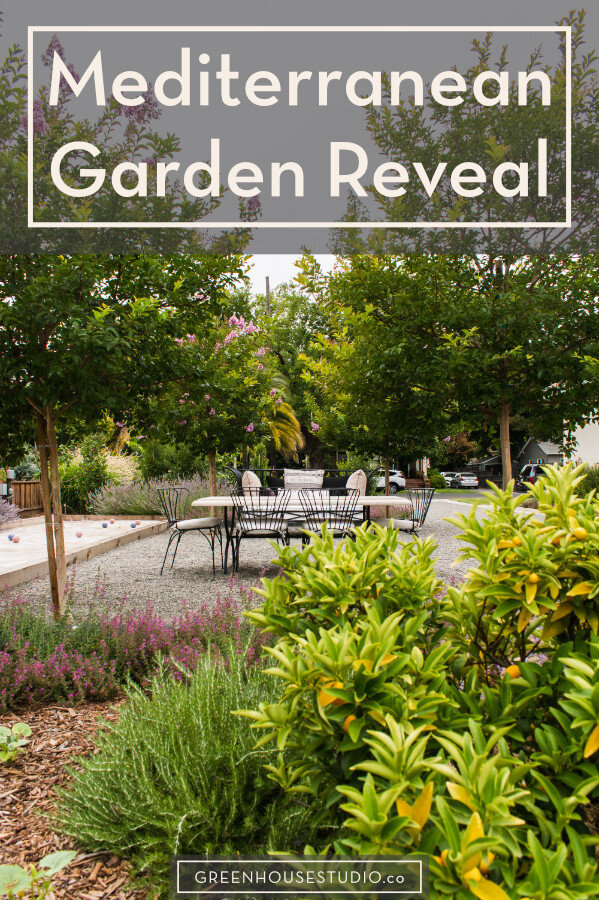This captivating photo, labeled "Mediterranean Garden Reveal" by GreenhouseStudio.co, showcases an elegantly designed backyard garden. The vibrant scene features a white table with matching chairs adorned with black wire frames and cushioned in white, set on a patch of silvery grass. Surrounding this seating area are a variety of plants, including light green bushes to the left with adjacent brownish mulch, and visually striking light purple plants, possibly lavender, nearby. Further details include spiky plants and an array of other lush greenery. The background reveals a suburban setting with visible cars, trees, another house, and possibly a street. The overall garden setting is intimate yet inviting, designed for leisure and social gatherings, adding to its enchanting suburban ambiance. The bottom of the image is branded with the distinctive GreenhouseStudio.co logo, suggesting this could be a front page of a magazine or an architectural mockup. The earthy tones—greens, yellows, pinks, and browns—are meticulously arranged, creating a harmonious and vibrant outdoor space.